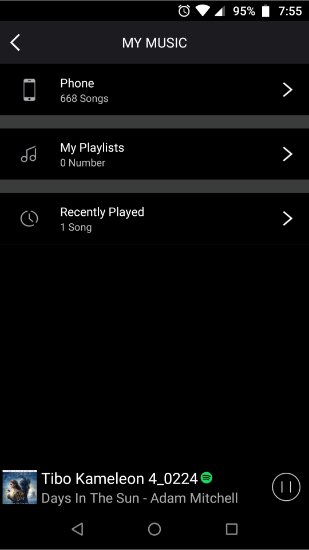This image captures the "My Music" section of a mobile music application titled "My Music." The user's phone displays a total of 668 songs stored. There are no playlists, and the recently played section includes just one song. Currently playing is "Days in the Sun" by Adam Mitchell. The device in use is the Teebo Chameleon 4_0 2 2 4. The interface shows playback controls with a small thumbnail of the album art, the title, and the artist's name, alongside a play/pause button. A small Spotify logo is also visible. Additional information includes a battery percentage of 95%, the current time (7:55), signal strength, and other standard icons. The overall color scheme is dark mode, featuring black and gray tones with white text for enhanced visibility.